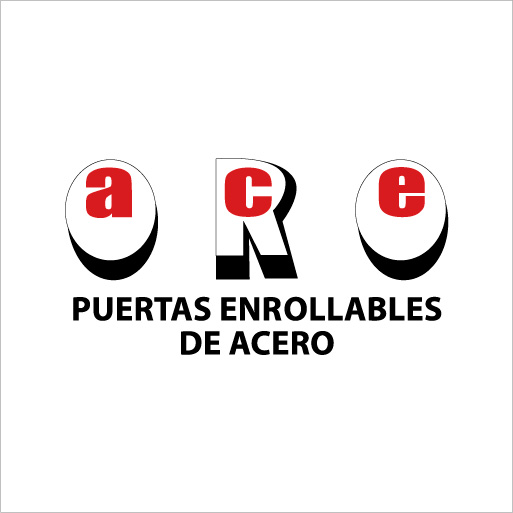The image features a logo with a white background and a thin black-lined square framing the design. Prominently centered are the three lowercase letters "a," "c," and "e" in a bright, eye-catching red. Each red letter is positioned against a semi-transparent, three-dimensional letter that creates a distinctive backdrop: the letter 'A' sits on top of an 'O,' the 'C' on top of an 'R,' and the 'E' on top of another 'O,' all of which have black drop shadows adding depth.

Beneath this main text, in bold, black capital block letters, the phrase "PUERTAS ENROLLABLES DE ACERO" is displayed, indicating a likely Spanish context referring to steel roll-up doors. The font used for the semi-transparent letters behind 'ACE' has a vintage 1960s style, enhancing the overall retro aesthetic of the logo.